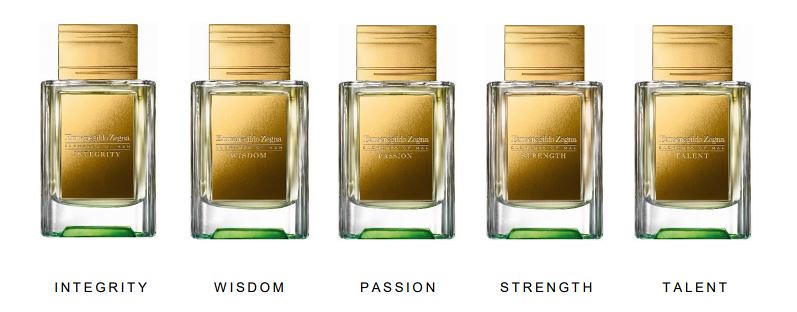The image shows five horizontally aligned shot glass-like containers, each with a clear, circular body and distinctive green bases. The containers appear identical, uniformly arranged in a neat row with no distinguishing background, highlighting their meticulous alignment. Each container holds a golden, bar-like object, possibly chocolate bars wrapped in smooth gold foil, stamped with what could be a brand name. The tops of these bars protrude from the containers. Subtle horizontal indentations are visible on the right and left sides of the image. Below each container, there are words in bold capital letters: "INTEGRITY" under the first, "WISDOM" under the second, "PASSION" under the third, "STRENGTH" under the fourth, and "TALENT" under the fifth.